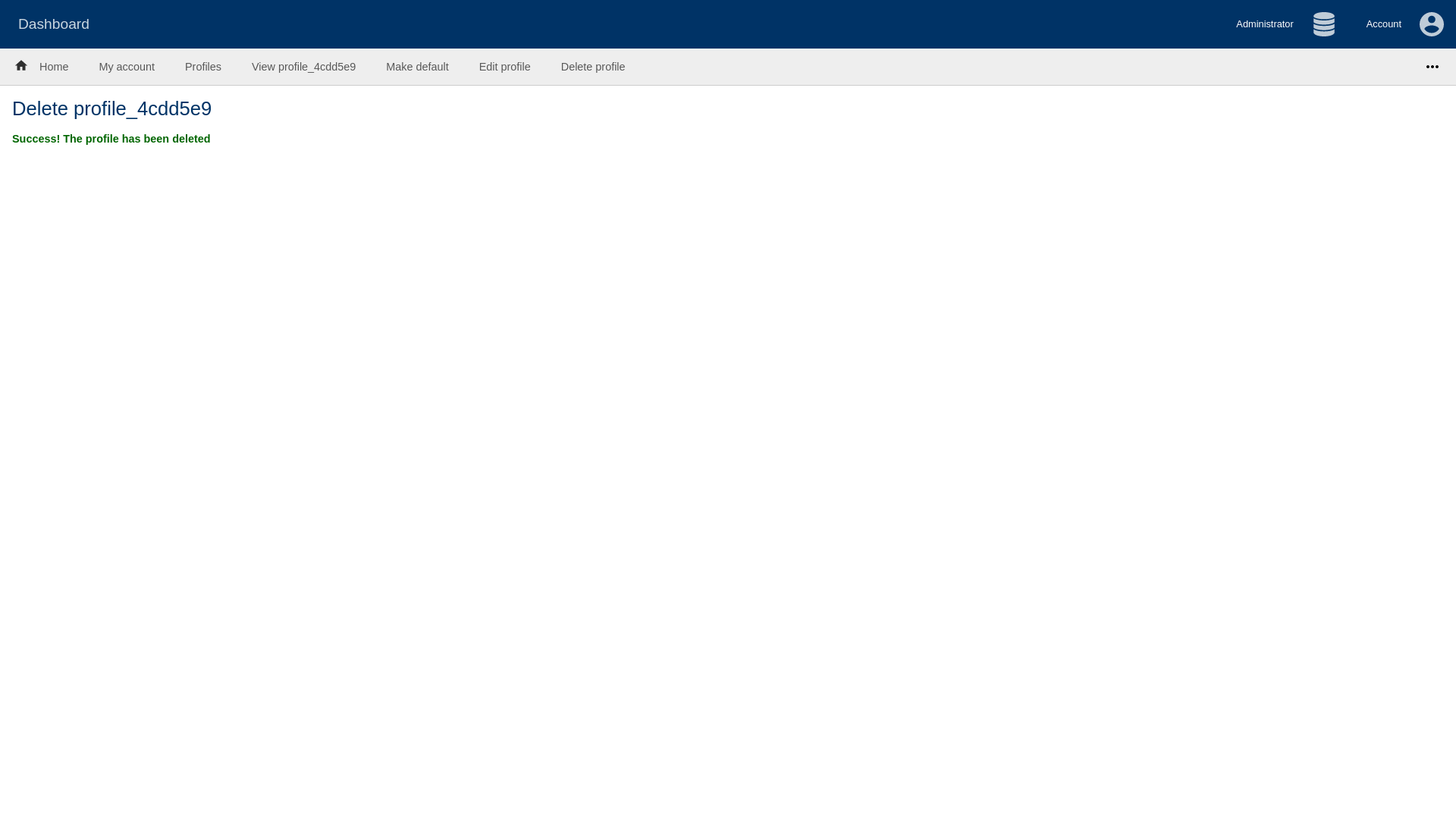Here's a detailed and cleaned-up caption for the provided image:

---

The screenshot displays a user's dashboard interface. Dominating the top of the page is a long blue banner. On the left side of the banner, the white text reads "Dashboard." To the right, the text "Administrator" is flanked by an icon resembling a stack of four coins. Further to the right, "Account" is visible, accompanied by a round gray icon featuring a blue human figure in the center.

Beneath the blue banner, a long horizontal gray line spans the width of the page. On the left side of this gray banner, there is a black house icon followed by "Home," "My Account," "Profiles," "View Profile under bar CDD5E9," "Make Default," "Edit Profile," and "Delete Profile." On the far right edge, there are three dots aligned horizontally.

Below this gray bar, the background turns white. On the left side, "Delete Profile under bar 4CDD5E9" is displayed in blue font. Beneath this, a green message reads, "Success, the profile has been deleted."

---

This caption provides a clear and detailed description of the dashboard interface elements.